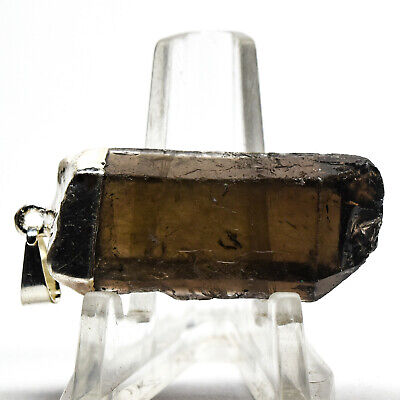The image prominently displays a close-up of a unique piece of jewelry, likely a pendant, resting on a clear acrylic stand. The central object is a semi-translucent, dark brown gemstone with a somewhat rectangular shape that tapers and becomes jagged on the right side, typical of faceted gems. On the left side, a gold hoop is affixed to the top, accompanied by a small diamond stud, suggesting the item might be an earring or charm. The gemstone appears to be set into a metallic silver backing, enhancing its intricate design. The clear acrylic stand beneath the gemstone slopes downward, cradling the gem securely. The entire setup is captured against a solid white background, with a light gray shadow subtly defining the stand’s base, enhancing the elegance and clarity of the display.